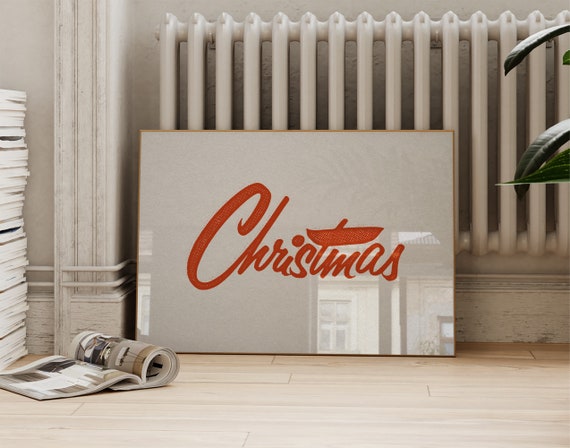In the photograph, a prominent glossy panel with a thin metallic frame takes center stage. The panel is predominantly beige and features the word "Christmas" in vivid red, handwritten-style letters. This panel leans against a white radiator, which appears to need a fresh coat of paint. The room is mostly white, with a clean, light beige wooden floor reflecting elements of the room.

To the left of the panel, an open magazine lies on the floor beside a tall stack of additional magazines. On the right side, a few leaves from a house plant are visible, slightly encroaching into the frame. The background includes a faint shadow of a plank and the room's overall minimalist décor enhances the focus on the festive message of "Christmas" in the foreground.